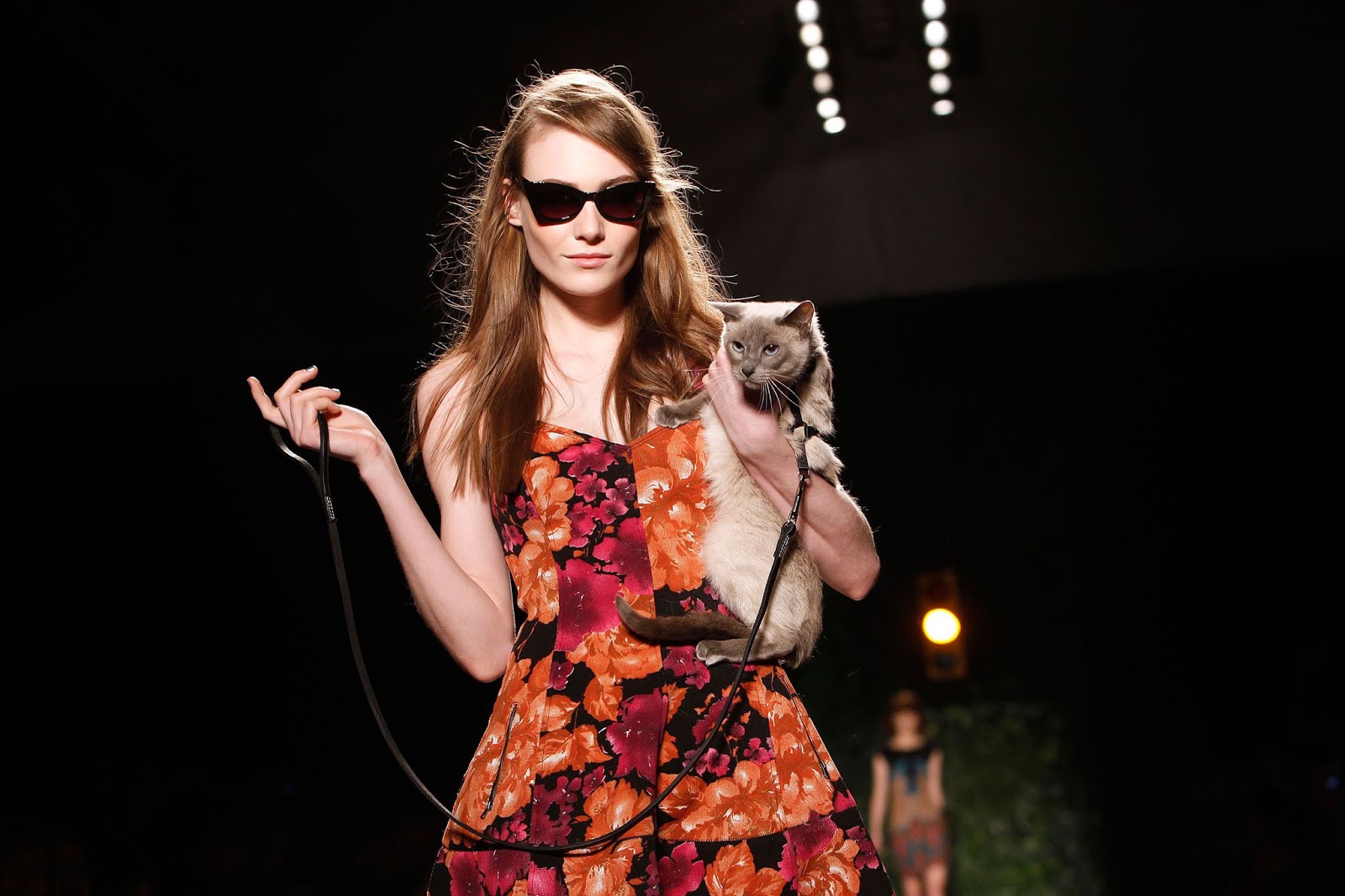In this striking photo, a poised woman, possibly a runway model, exudes elegance and confidence. She is clad in a chic dress adorned with intricate floral designs in vivid shades of lava pink and blood orange that stand out vividly against the black backdrop of the fabric. Her sophisticated look is accentuated by a pair of stylish glasses. The model holds a light tan cat on a leash in her left hand, suggesting that it's her pet. The cat's relaxed demeanor contrasts with the high-energy environment, creating an intriguing dynamic in the image. In the background, another model, slightly blurred to emphasize depth, waits her turn, hinting that they are on an elevated platform, likely part of a fashion show runway. The main model's position indicates she might be at the end of the runway, about to do the classic end-of-runway twirl before heading backstage, where the next model will soon follow.